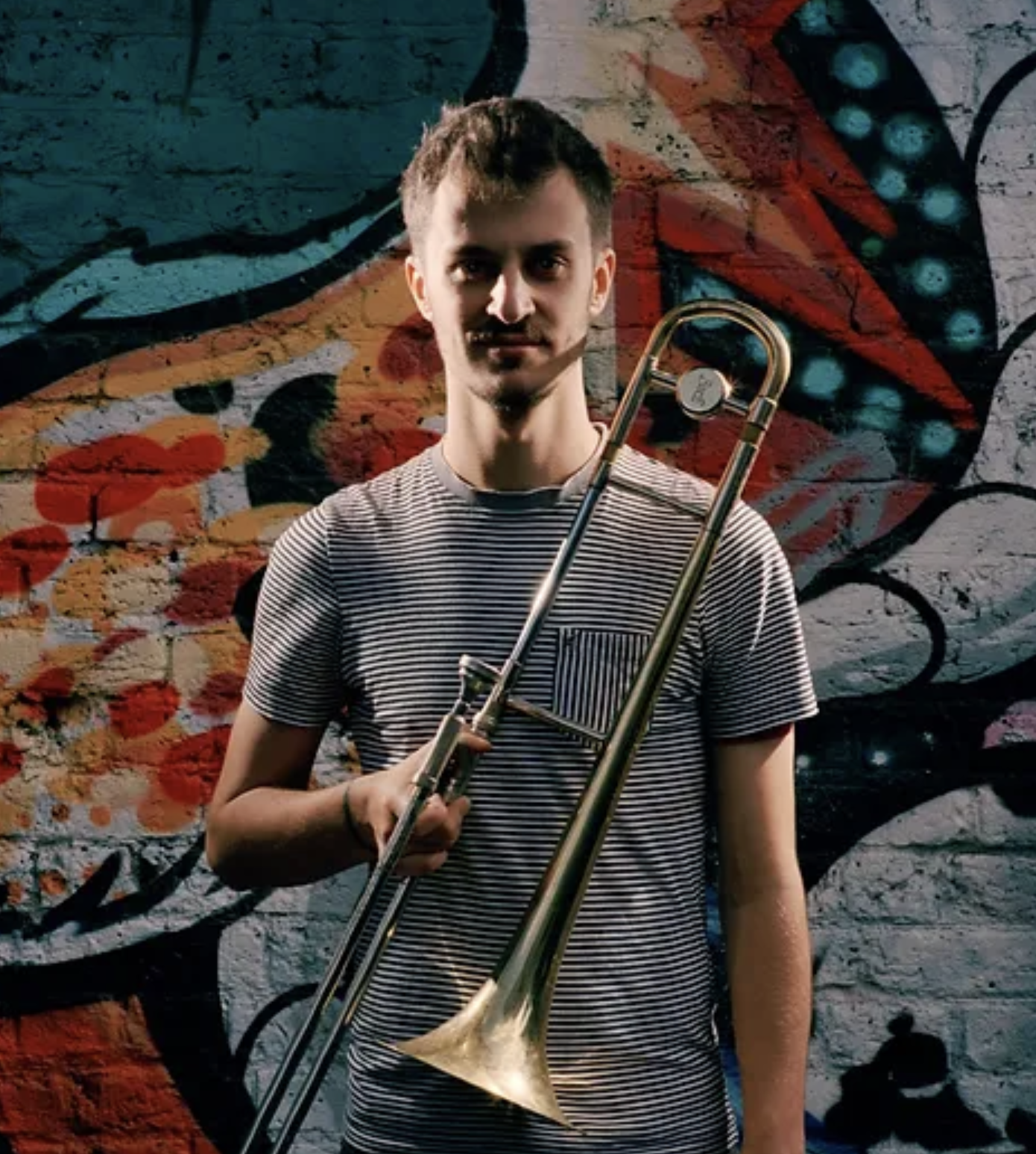A man with light brown, somewhat messy hair, and a neatly kept mustache and goatee stands against a vibrant mural-covered brick wall. His hair falls over his forehead and is clipped close on the sides. The mural is a riot of colors, featuring green, light green, red, and orange blotches, with blue circles in the upper right corner, all set against a white and black backdrop with various abstract designs. The man is dressed in a tightly-fitted, short-sleeved black and white horizontally striped t-shirt, which also has a vertical striped pocket. He holds a brass trombone in his left hand; the instrument’s bell hangs down past his stomach while the top curves over his right shoulder. His right arm hangs straight down by his side and extends out of the frame. An intriguing shadow casts across his face, created by the ambient light.